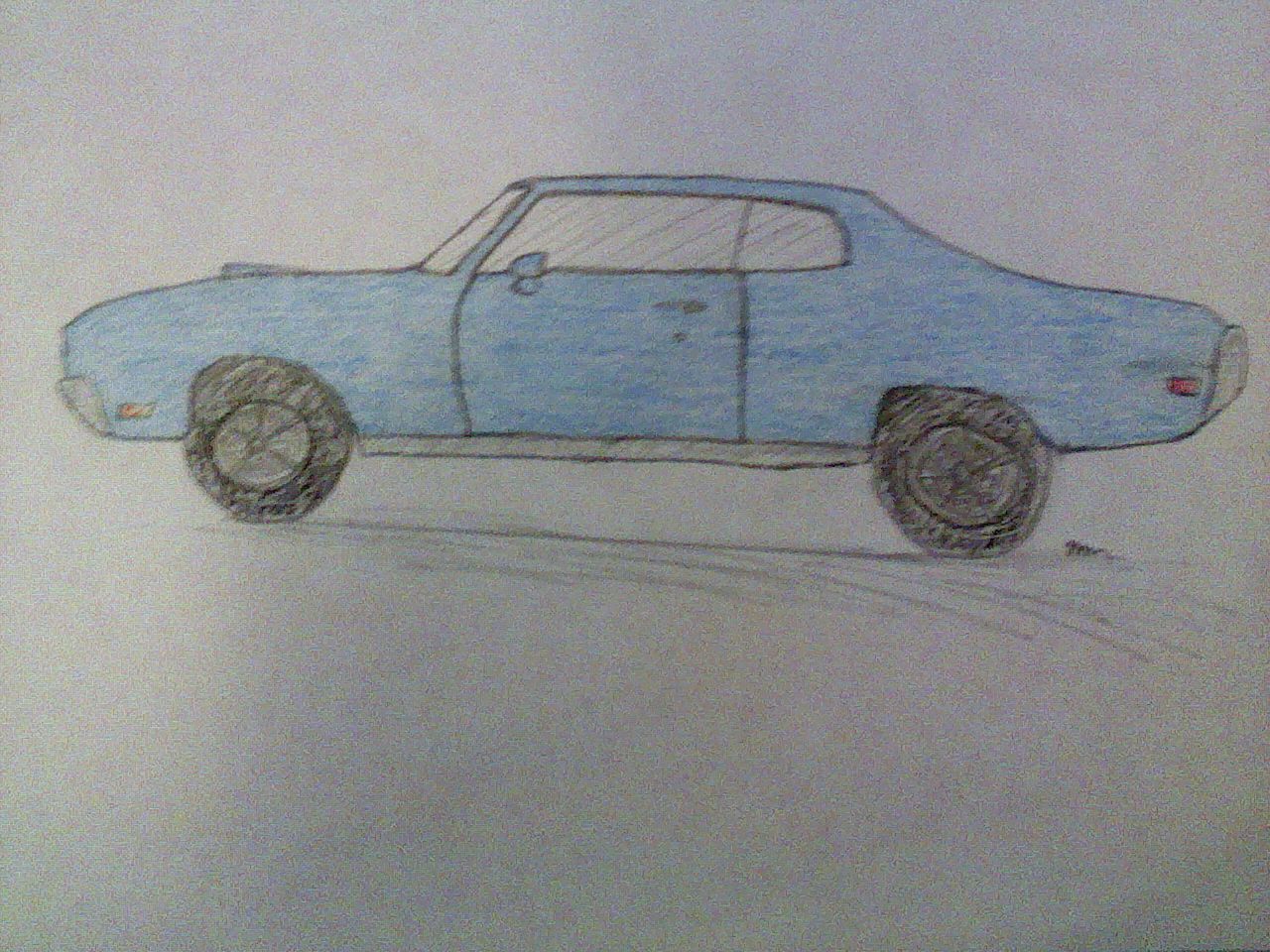This image captures a child's drawing of a blue sports car in motion. The car, rendered in crayon with pencil-like outlines, is driving to the left on a white background. The vehicle has black, solid-colored tires with penciled-in tire marks beneath them, adding a touch of realism. Detailed features include tinted windows, a noticeable engine air intake bump on the hood, and blinkers—one yellow in the front and one red in the back. The car is a two-door model, with a visible driver's side door and a small side mirror. The drawing, while not highly artistic, effectively uses pencil and crayon to create distinctions between the car's body and its windows and doors, accented by black outlines. The addition of squiggly lines below the car suggests motion and a shadow, enhancing the dynamic feel of the image.